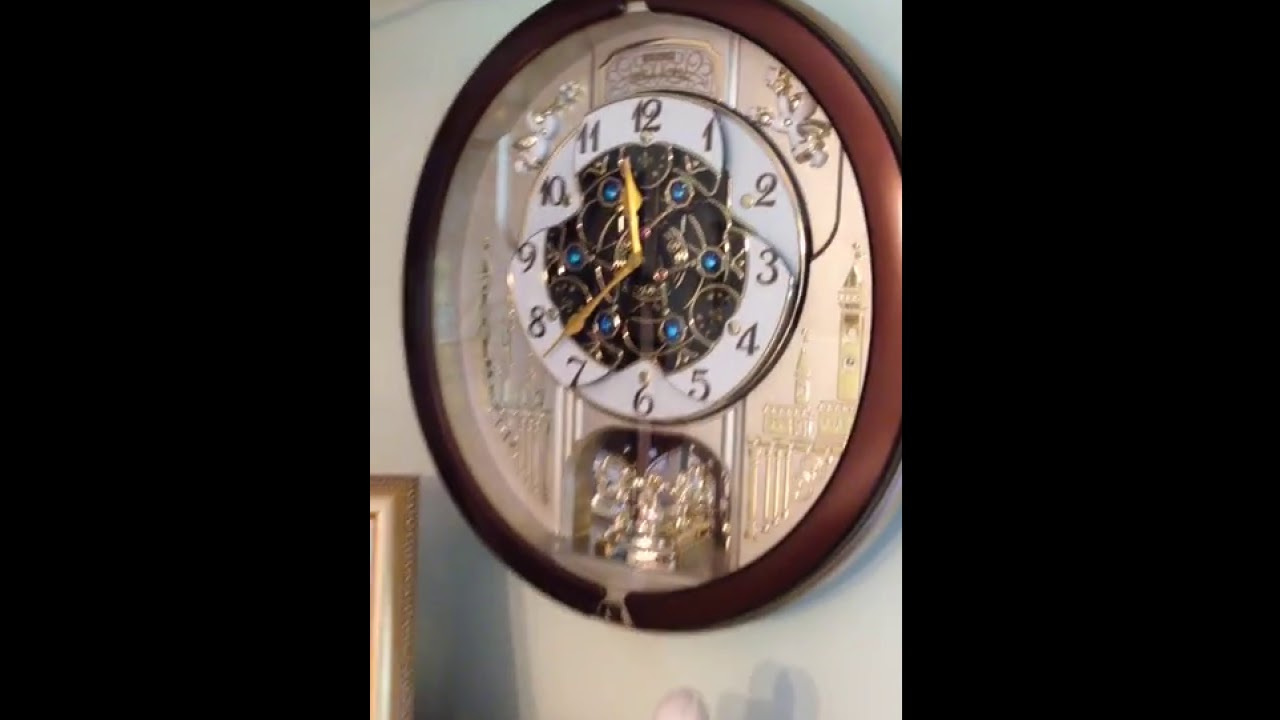The horizontally aligned, rectangular image showcases a vertically oriented, ornate round clock mounted on a slightly blurry white wall. This image, framed by thick black borders on either side, highlights the centerpiece: a clock with a glossy brownish-red rim encasing a white clock face adorned with gold embellishments. The clock numbers, ornately written in dark brown, circle the face which is further accentuated with blue gems connected by gold wires. The clock hands, in gold, point to numerals set within a decorative bezel. Below the clock face, a section showcasing intricate mechanisms and additional decorative elements is visible. The image's upper left-hand corner and bottom portion are particularly blurry. In the lower left-hand corner, part of a gold-framed picture is partially visible, adding context to the surroundings of this striking timepiece.